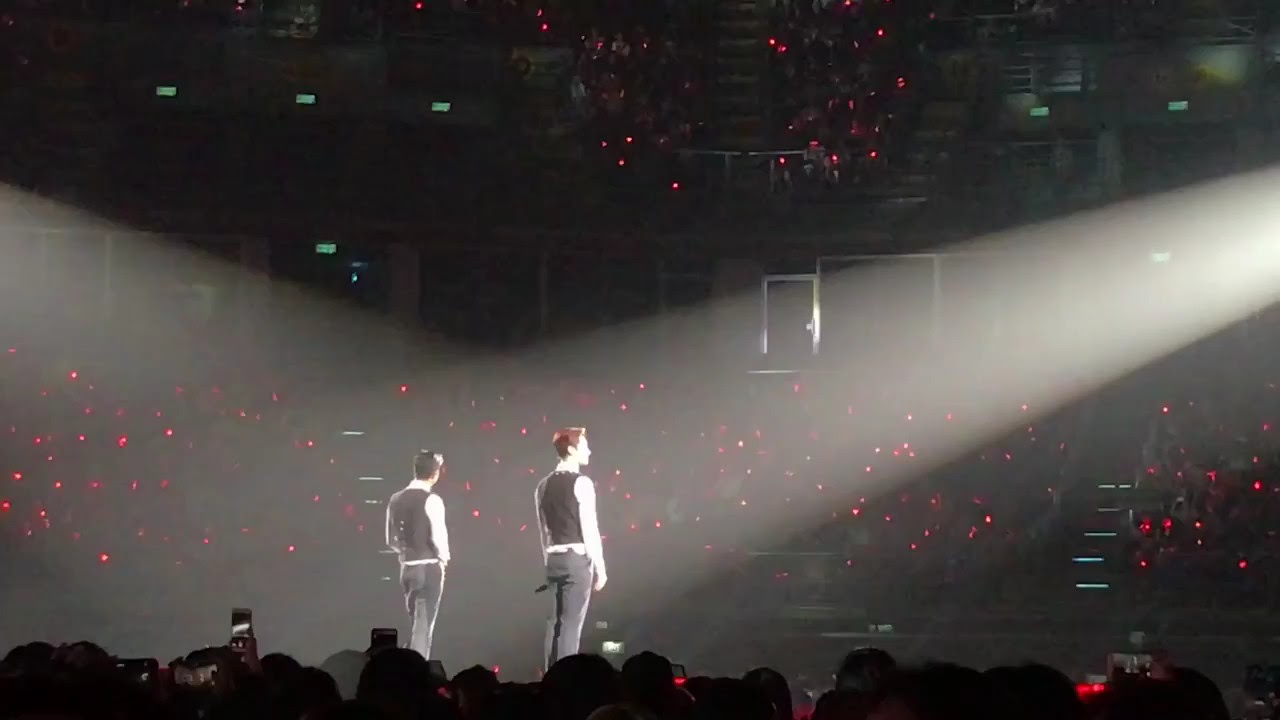The image depicts a pixelated photograph of two young men standing on a stage, facing a large audience. Both men, one with dark brown hair and the other with slightly lighter, reddish-tinted hair, are wearing matching outfits: white button-down shirts with black vests and gray dress pants. Their backs are turned to the camera as they hold microphones, positioned slightly to the right of center stage. The crowd appears to be illuminated by numerous red lights and other colored dots, likely from the cell phones of the spectators who are capturing the moment. The venue is shrouded in darkness, with only two white spotlights from either side and multiple overhead stage lights illuminating the performers. The audience, whose faces can't be distinguished due to low image quality, encircles the stage in what looks to be a packed arena, adding to the atmosphere of the concert or event.